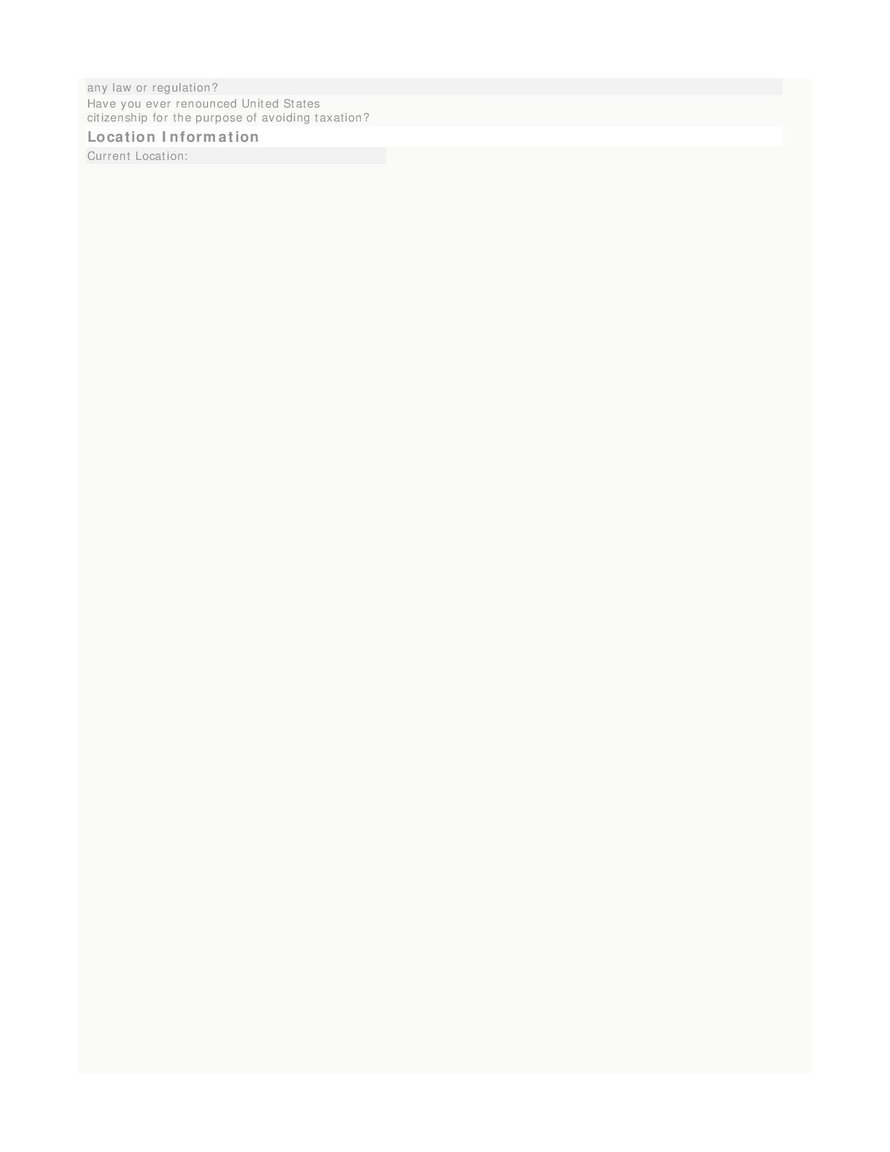The image depicts a portrait-oriented screenshot featuring text on a predominantly white background. At the very top, a greyish bar contains the question, "Any law or regulations?" Below this, another line reads, "Have you ever renounced United States citizenship for the purpose of avoiding taxation?" Directly beneath this query, a bold white bar displays the heading "Location Information." Following this, a smaller greyish bar lists "Current Location," although no specific information is provided next to it. The text occupies only a small portion, approximately an inch, of the image's upper section, leaving the rest blank and devoid of additional content.